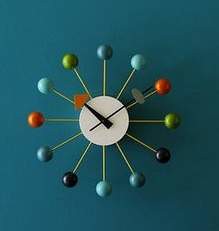In this image, a uniquely designed clock is set against a solid blue-green background. The clock features a minimalistic white center with thin, black hands. The minute hand ends in a gray ball, while the hour hand terminates in an orange triangle. Surrounding the white center, twelve sticks radiate outward like spokes, each topped with a colorful ball. The balls come in a variety of colors: green, blue, red, black, and turquoise. This modern, numberless design relies on the colorful sticks and balls to resemble the positions of traditional clock numbers, creating a vibrant and eye-catching timepiece.